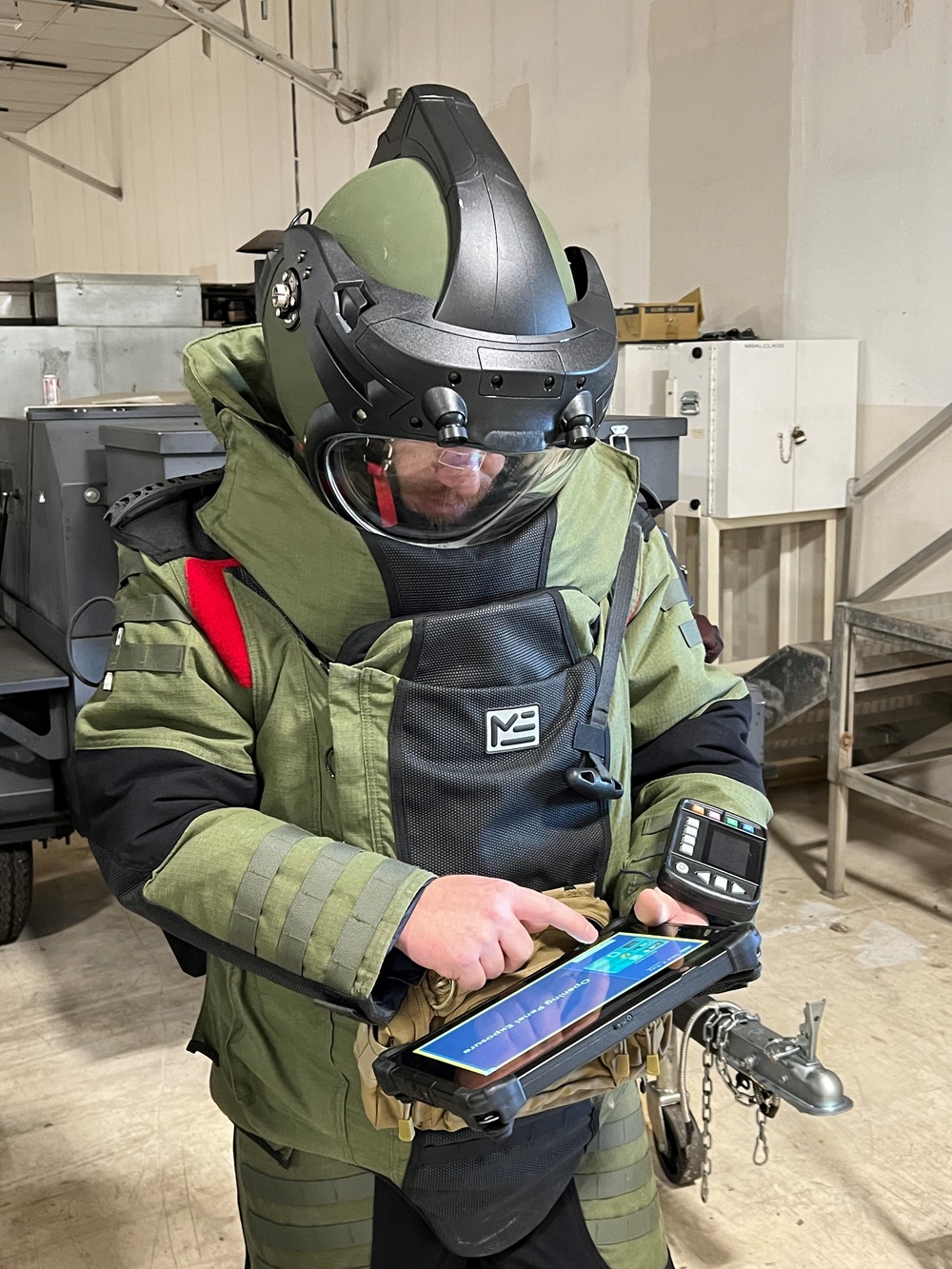In the center of the image, there is a man wearing a bomb diffuser suit, characterized by its thick, greenish-black padded fabric designed to provide protection in hazardous situations. The suit covers his body from head to the top of his upper legs, leaving only his hands exposed as he operates a heavy-duty iPad. His helmet is substantial and features black and green colors, equipped with lights resembling microscope-like structures, and a glass shield over his face. On one of his sleeves, a computer device is visible. He stands in an industrial setting, filled with various machinery and technical equipment, against a backdrop that includes a poured concrete floor and a trailer-like structure. The environment suggests a high-risk area where specialized protective gear is essential.